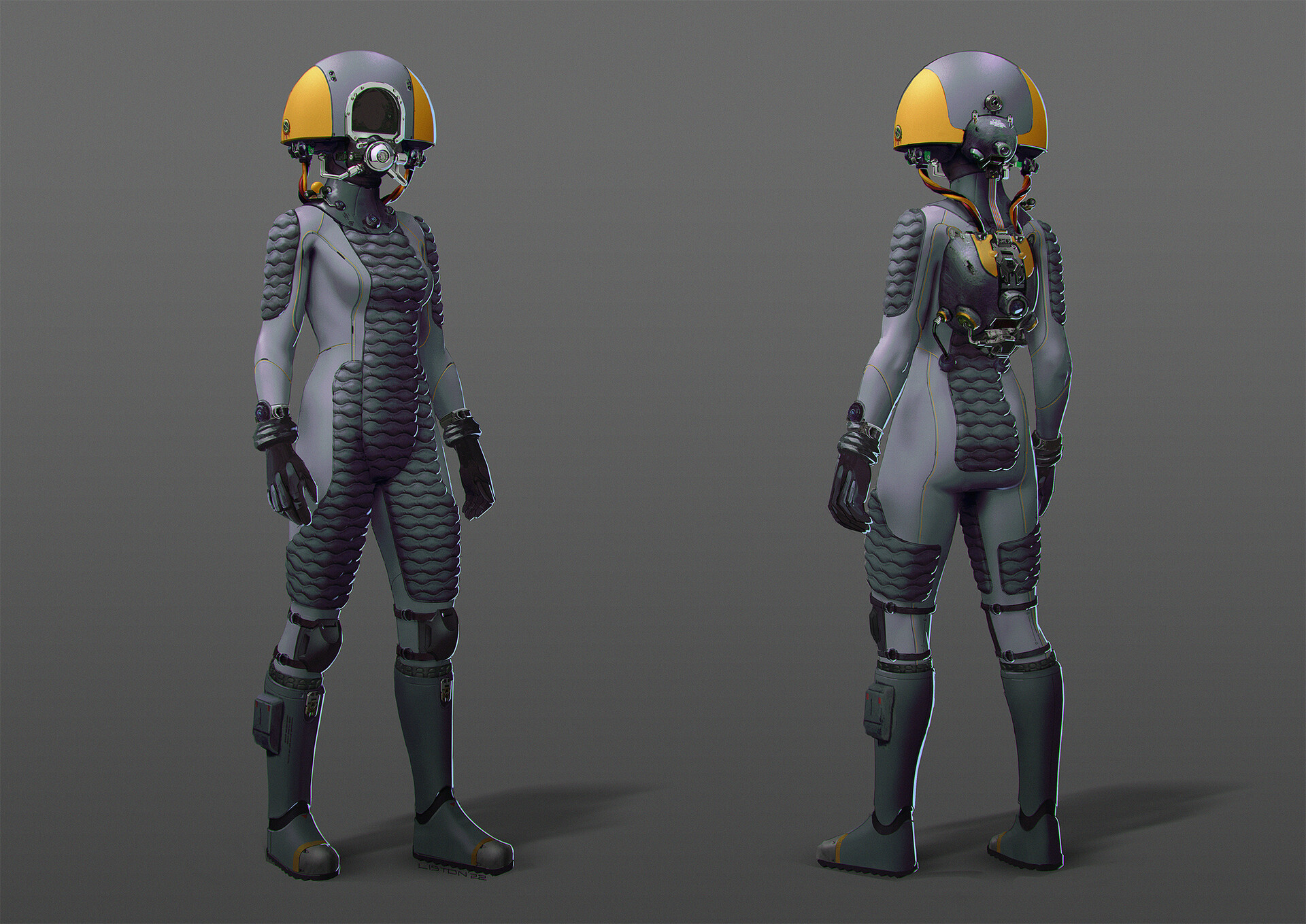This image showcases two futuristic female astronauts or space travelers, both clad in detailed protective suits. The background is a subtle light gray, providing a neutral setting to highlight the intricacies of the outfits. The figure on the left is depicted from the front, facing right, while the figure on the right is shown from the back, facing top-left.

Each astronaut is dressed in a form-fitting, purple-gray suit accented with black trim and knee-high black boots. Black gloves and knee pads enhance the protective appearance of the ensemble. Their unique helmets feature a crescent or half-moon shape, with gray and yellow coloring, and they include a darkened glass window in the center for visibility. A circular silver mouthpiece and attached backpack-like structure, presumably for oxygen, complete the high-tech look of these suits. The careful positioning of the figures—one showing the front and the other the back—offers a comprehensive view of their gear, emphasizing their potential role as space travelers or astronauts.